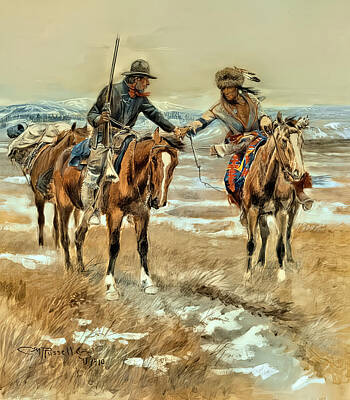This painting portrays a dramatic scene featuring two men on horseback in a vast, golden grassy field interspersed with patches of melting snow. In the background, snow-capped hills and mountains rise under a dull gray, cloudy sky. The central figures are a cowboy and a Native American, each atop brown and white horses that face towards the viewer.

On the left is a cowboy in a dark gray hat, long-sleeve blue shirt, light-colored pants, and boots, with a bandana around his neck. He grips a rifle in his right hand while extending his left to clasp the hand of the Native American. His horse has a rich mocha brown hue with a distinctive white stripe running down its face. There is also a blue blanket visible under his saddle, and behind him is a pack horse carrying goods wrapped in white blankets.

To the right is the Native American, adorned in a fur cap with feathers. He sports a light-colored top and rides a lighter beige horse, which has a multicolored blanket under its saddle. Both men, appearing to have tanned skin, share a moment of connection in this tranquil yet striking landscape.